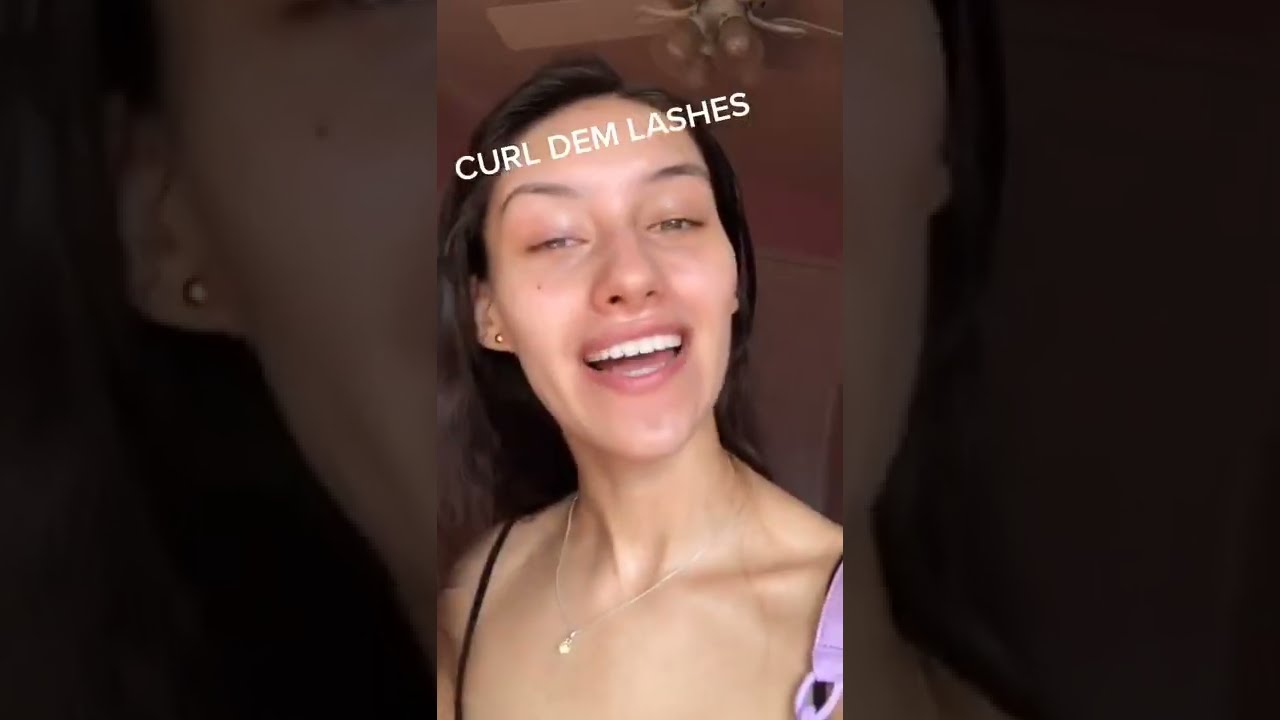This vertically-oriented photograph, taken likely with a cell phone, features a close-up of a young white woman with very fair, smooth skin and mid to long dark brown hair. The image showcases her head, neck, and upper shoulders, with a repeating, darker version of the same image filling the background. The focal point is the central vertical rectangle where the main photograph resides. The woman is smiling broadly with her mouth open, as if mid-conversation, revealing her very straight, white teeth. Her eyes are slightly squinted, giving her a joyful, expressive look, although her right eye seems slightly affected, possibly hinting at irritation or swelling. She has brown eyes and well-defined, thin arched eyebrows. The woman is accessorized with small gold stud earrings, a delicate necklace featuring a small pearl pendant, and a light lavender strap over her right shoulder, likely part of her outfit. She's wearing a spaghetti strap tank top possibly with black straps. Above her forehead, there is a prominent white text in all capital letters saying "CURL DEM LASHES," hinting at a possible beauty or makeup context. She appears to be indoors, possibly in a room within a house.